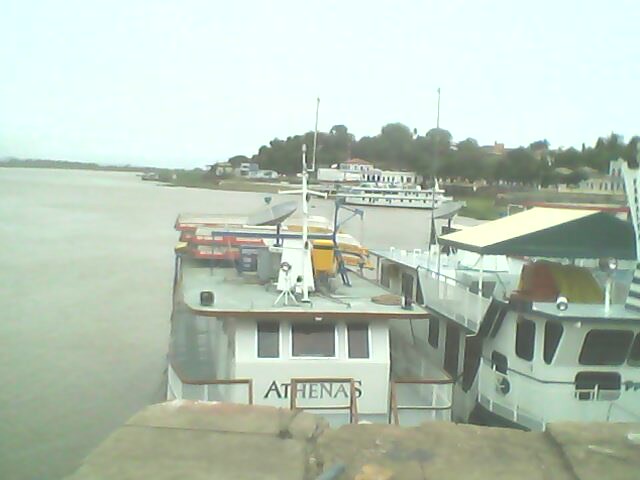This image captures an atmospheric scene of a waterway, possibly taken years ago given the old-fashioned appearance. It features two prominent white party boats, one named Athena’s, which anchor side-by-side along a stone wall. Athena’s boat is easily recognizable, partially due to its green roof and large windows. The boats are set against a backdrop of a cloudy, overcast sky that casts a grayish hue on the water. Surrounding the mooring area are decks or slabs, possibly used for boarding. Further into the distance, the image reveals an array of tall trees and various buildings, including houses lining the shoreline. There’s also a partial view of a bridge spanning over one of the boats. The composition, dominated by various shades of gray and green, conveys a serene yet somewhat somber ambiance, indicative of an older photograph.